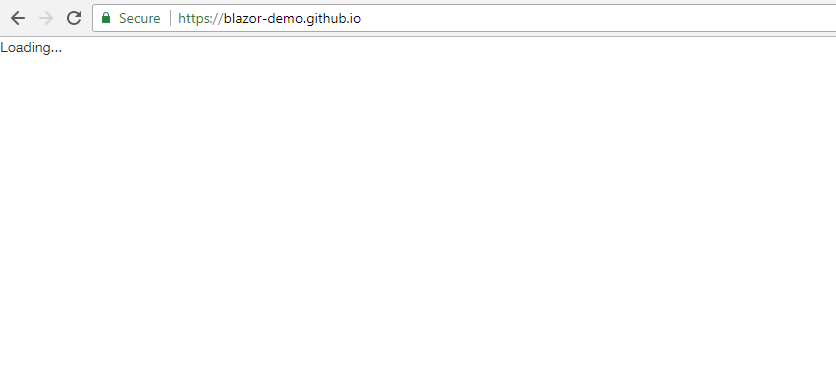The image captures the top section of a computer's web browser interface. At the very top, there is a long, skinny, gray rectangular bar. Within this bar, on the left side, there are navigation buttons: a dark, prominent left-pointing arrow, and a faint right-pointing arrow, indicating that the left arrow has been recently clicked. 

Next to these arrows, there is a refresh button, symbolized by a circular arrow, suggesting that the page can be reloaded. Adjacent to the refresh button is a white rectangular address bar that contains a black padlock icon followed by the text "Secure." The bar then displays the URL "https://blazor-demo-github.io". 

Directly beneath the address bar, a status message reads "Loading..." indicating that the page's content is currently still loading. The rest of the screen below this message is completely blank, with no text, images, or other content visible.